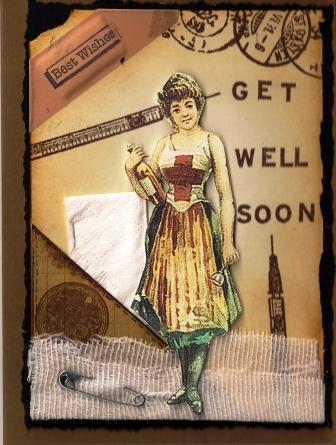The image presents a vintage-style postcard or poster with a sepia-toned background. At the top left corner, "Best Wishes" is inscribed, while at the top right, there are three coin-like circles with various writings and some postmarks. Below the postmarks, the words "Get Well Soon" are prominently displayed in brown capitals. A syringe can be seen emerging from the left side and another from the bottom right corner. Across the bottom of the image, gauze fabric, held together by a safety pin, stretches horizontally. In the center stands a charming woman with blonde hair styled back, wearing a white tank top adorned with a red cross and a combination of a green knee-length skirt and a yellow apron. She holds a bottle of wine in her right hand and a glass of wine in her left hand, completing the intriguing blend of medical and celebratory elements in this visually compelling scene.